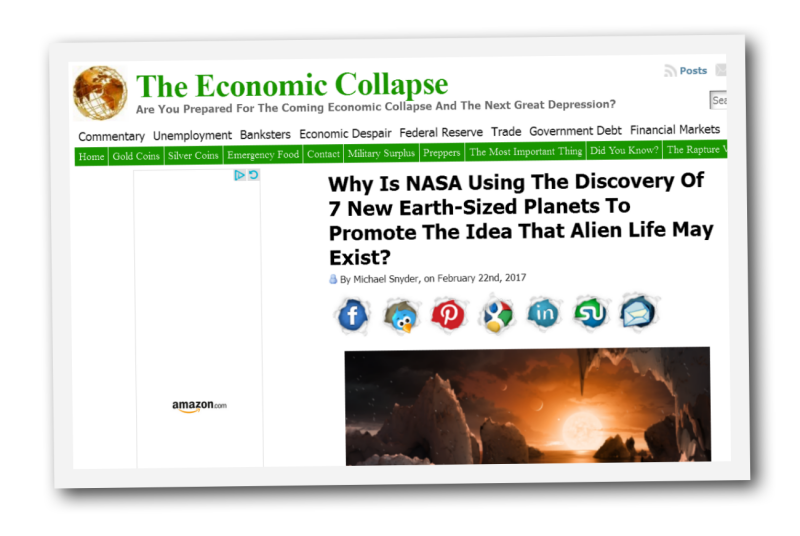The image is categorized under "website." It features a wireframe globe adorned with gold continents at the top, set against a white background. Large green letters spell out "The Economic Collapse" across the top. Below this, in slightly smaller letters, it reads, "Are you prepared for the coming economic collapse and the next Great Depression?" 

Further down, a series of keywords are displayed: "Commentary, Unemployment, Banksters, Economic Despair, Federal Reserve, Trade, Government Debt, Financial Markets." 

Directly beneath this section, green boxes with white text offer navigation options: "Home, Gold Coins, Silver Coins, Emergency Food, Contact, Military Surplus, Preppers, The Most Important Thing, Did You Know, and The Rapture."

At the very bottom, it states, "Why is NASA using the discovery of seven new Earth-sized planets to promote the idea that alien life might exist?" 

Clickable icons for Facebook, Twitter, Pinterest, and Google are also present.